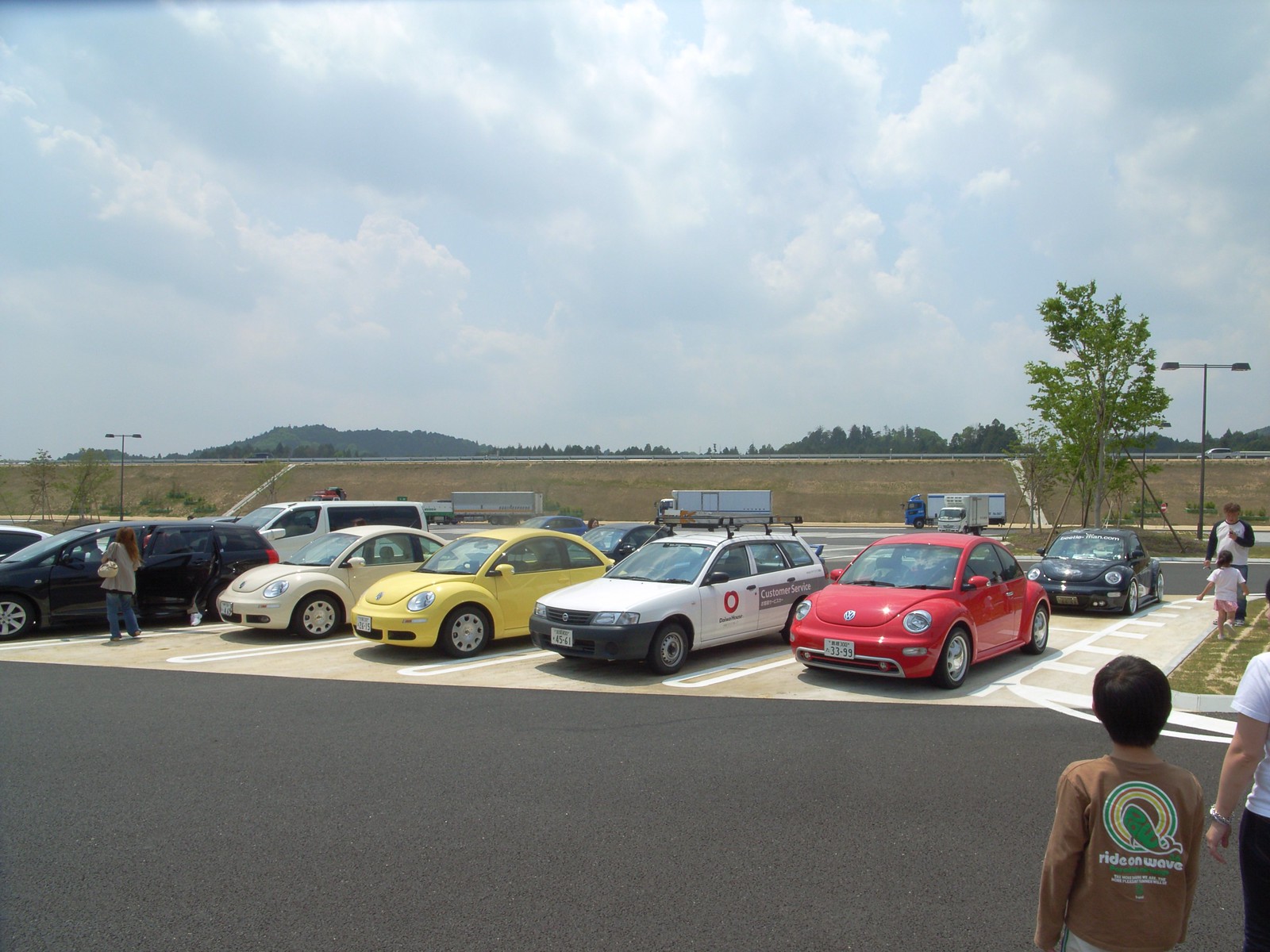This photograph captures an exterior scene dominated by a spacious, light-colored concrete parking lot. The parking spaces are angled, housing a variety of vehicles, including a distinctive array of Volkswagen Beetles in red, yellow, white, and black. In the foreground, a child wearing a brown shirt with a whale emblem stands with a parent on the right-hand side. The midground features a broad driving lane within the parking lot, leading up to a set of trucks traveling on an interstate road that runs parallel to the parking lot. The horizon reveals green hills and trees beneath a blue, cloudy sky. A noticeable detail is a hill supporting the interstate, with cars moving along it and a railing visible. In the background, a large, well-braced young tree marks the scene's edge. Pedestrians, including a woman, a boy, a man, and a girl, are seen moving about, contributing to the activity typical of an American parking lot.